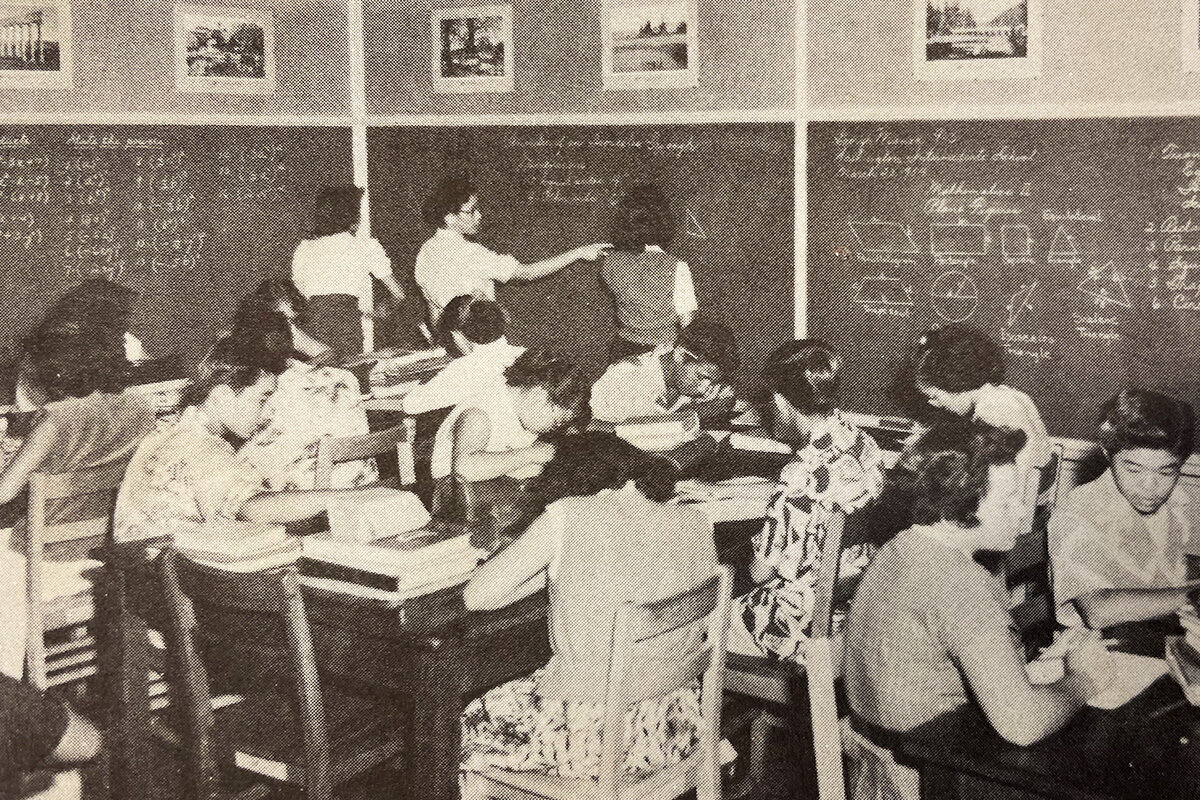This is a black and white photograph depicting a vintage math classroom, likely from the 1950s or earlier. In the foreground, there are three wooden tables, each seating six students who are intently poring over their textbooks or engaged in quiet discussions. The students' period attire suggests a mid-20th-century setting. In the background, three chalkboards stretch across the width of the image. On the left chalkboard, algebraic equations are clearly visible, while the right chalkboard displays various geometrical shapes, including a rhombus, trapezoid, circle, and different triangles. The center chalkboard has cursive writing that is not clearly legible. Standing at the chalkboards are three individuals who appear to be teachers; one teacher points at another student as they write on the board. Above the chalkboards, the plain bordered section of wall is adorned with photographs or paintings of Roman arches and other architectural landmarks. This detailed and historically rich scene captures the essence of mid-century educational environments.